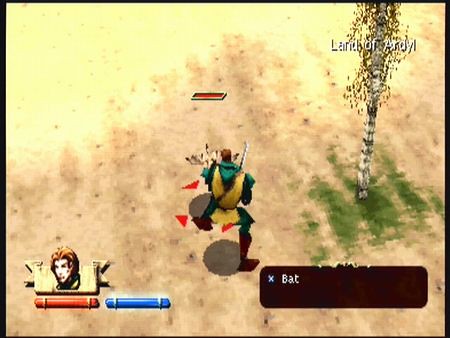This color photograph, evocative of a video game screen with simple, pixelated graphics, features a predominantly yellowy-beige background that transitions from pale yellow in the upper left to a brownish beige towards the middle and bottom, suggesting a ground surface. A narrow black border encircles the image, hinting at a mobile or retro console display.

Central to the scene is an avatar in a green and yellow tunic or uniform, facing away from the viewer, with circular shadows beneath their feet and red triangles around the left foot. Above the avatar's head, there is a small red rectangle. To the right stands a tree, resembling a birch tree with a white and brown trunk and green grass beneath it. Words are printed on the tree branches, partially obscured but reading "Land of Ardill."

In the bottom-right corner, there is a distinctive logo featuring a woman's face. Adjacent to this logo is a red and blue bar, and slightly to the left is a brown rectangle with rounded corners, a blue circle marked with a white X, and text that says "Bat."